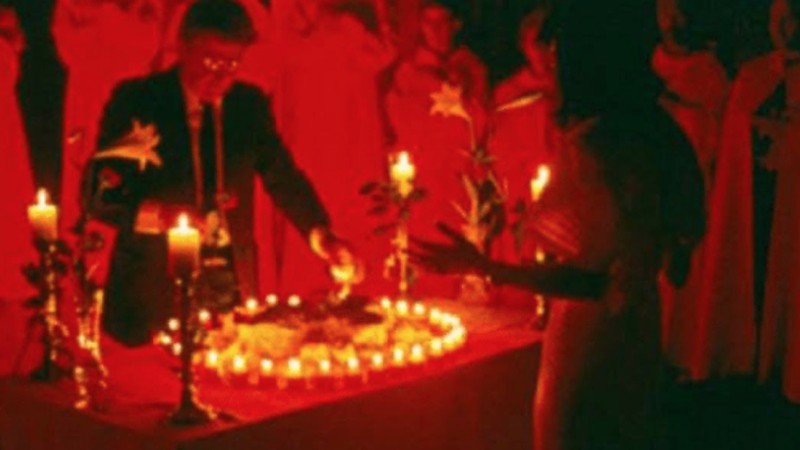The image depicts a low-resolution scene, set in a reddish-black hue, showing a group of people standing around a table adorned with numerous yellowish candles. The table features an elaborate candle arrangement, with four candles positioned at each corner and a cluster of candles at its center, casting a warm, light-yellow glow. This setup suggests a celebratory or commemorative event, possibly a wedding or a memorial service. The focal point is a man on the left, dressed in a black business suit with a tie and glasses, reaching over the table. Opposite him stands a woman in a formal dress, with long hair, although her face is not visible. Both the man and woman appear engaged in a ceremonial act, with the man seemingly lighting the central candles. The background hints at more individuals, adding to the atmosphere of a significant, perhaps ritualistic gathering.